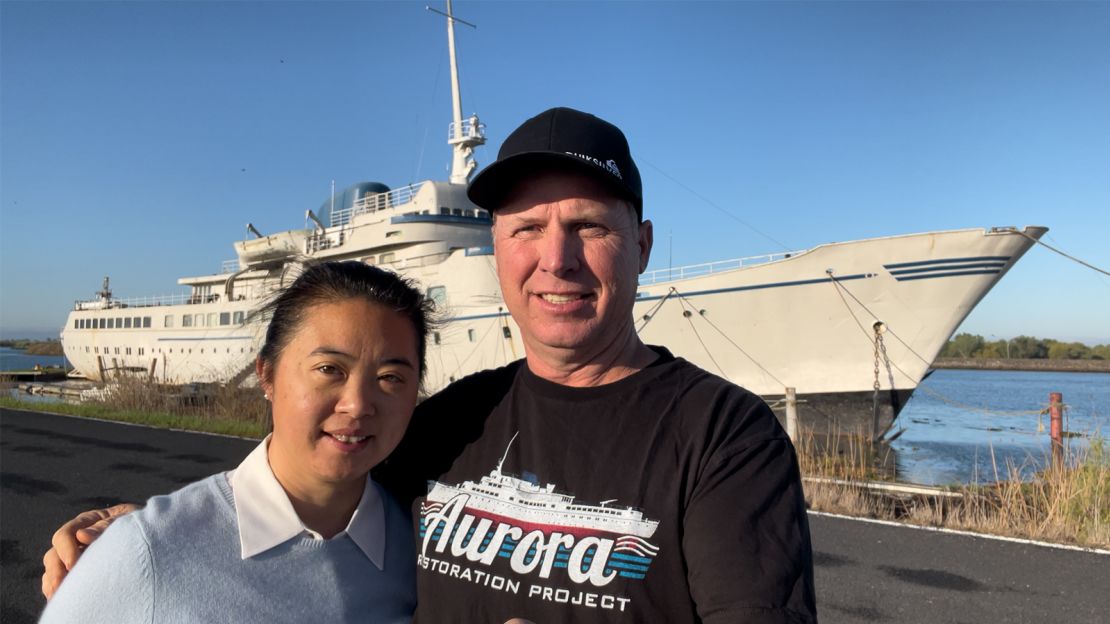This photograph captures a man and a woman standing on a road in front of a large white boat, which resembles a yacht or a battleship, with a rough appearance and three dark stripes at its front. The sky is bright and cloudless, suggesting a clear day, and beyond the boat, there's a grassy area and a body of water. The woman, of Asian descent, stands on the man's right and has her black hair tied back. She is dressed in a white collared blouse under a light blue sweater. The man, who is approximately a foot taller and appears to be Caucasian, wears a black baseball cap and a black t-shirt with a drawing of the boat along with the words "Aurora Restoration Project" and blue horizontal lines behind the word “Aurora.” Both individuals seem to be in their 40s or 50s, and the man has his arm around the woman, adding a sense of closeness to the scene.